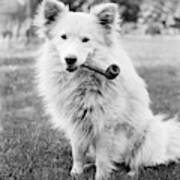A small, square black-and-white photograph captures a fluffy white dog with a serious expression, characterized by its small, dark eyes and black nose. This medium-sized, shaggy dog is seated on a mowed lawn, slightly turned to the left, displaying a thick, bushy tail that extends out of the frame to the right. The dog, facing directly at the camera, holds a large, thick-bodied pipe, carved from what looks like wood, that hangs from the left side of its mouth, over its shoulder. Its upright, triangular ears have a hint of dark color on the inside. The background, though indistinct, shows patches of grass and a faint line of trees or bushes along the upper edge of the image, with grass visible around the dog's front paws.